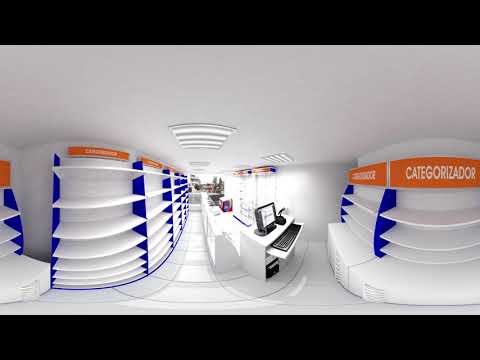The image depicts the interior of a bright, white-tiled room, possibly a small convenience store or storage area, completely devoid of products. The floor is covered with white tiles, and the walls and ceiling are similarly white, contributing to the bright ambiance. Dominating the space are large, empty shelving units characterized by their white shelves and distinctive vertical blue slats separating them. Each shelf unit has an upper section marked with an orange rectangular sign bearing white lettering; one such sign reads "CATEGORIZADOR," likely indicating organizational categories.

A central aisle leads to the back of the room, where a counter can be observed, although the specific items on this counter are indiscernible from the image. On the right side of the aisle stands a white counter equipped with a computer featuring a black monitor and keyboard, with the keyboard housed in a sliding drawer. Adjacent to the computer monitor is either a microphone or a scanner, possibly part of the store's intercom system. The background showcases more shelving and desks, further emphasizing an environment designed for business or storage purposes. The stitching effect appears to combine multiple angles into a single, comprehensive view, and notably, there are no people present in the image.